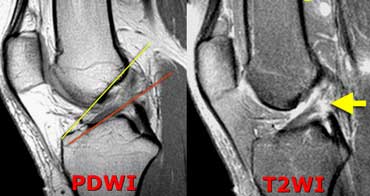The image presents two black-and-white scans, likely an MRI or x-ray, depicting cross-sections of a person's knee joint. Both scans, labeled PDWI on the left and T2WI on the right in red font, detail the same anatomical region but highlight different structures. In these scans, the knee joint is evident, identified by the presence of long bones and the curvature indicative of the femur and tibia, with cartilage appearing as white against the light gray bones. Surrounding muscles and ligaments are visible in darker gray tones. The left image features diagonal lines—one yellow and one red—pointing from the top right to the bottom left, indicating specific points of interest on the joint. Similarly, the right image includes a yellow arrow extending from the center right towards the image's center, emphasizing another anatomical detail.